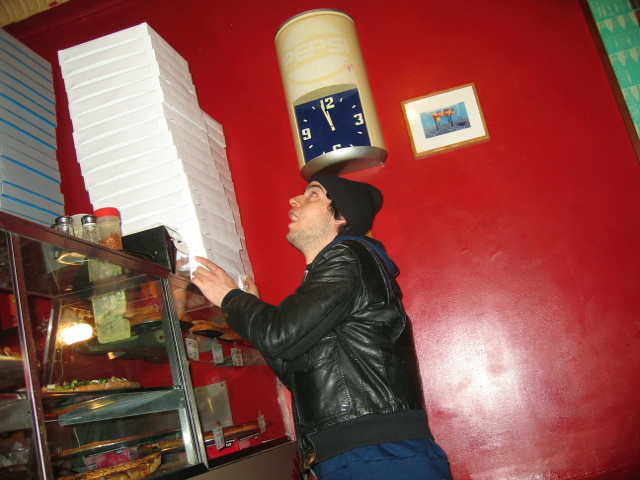In the photograph, a man stands in the foreground within a pizzeria, drawing attention as he gazes upward with his mouth slightly open, possibly examining a menu on the wall. He sports a black leather jacket, blue pants, and a black beanie, with dark hair peeking out. The backdrop features a vibrant brick-red wall adorned with a distinctive Pepsi clock that resembles a can, displaying the time as 11:58. A partially obscured photograph with indistinct figures adds to the wall's decor.

The man is positioned in front of a glass display counter showcasing an array of pizzas on various tiers. White pizza boxes are stacked on and around the counter, and a napkin holder is visibly perched atop it. The counter also holds several spice shakers, including jars of crushed red pepper, salt, pepper, and possibly grated Parmesan cheese. No employees are visible behind the counter, leaving the pizzas unattended.